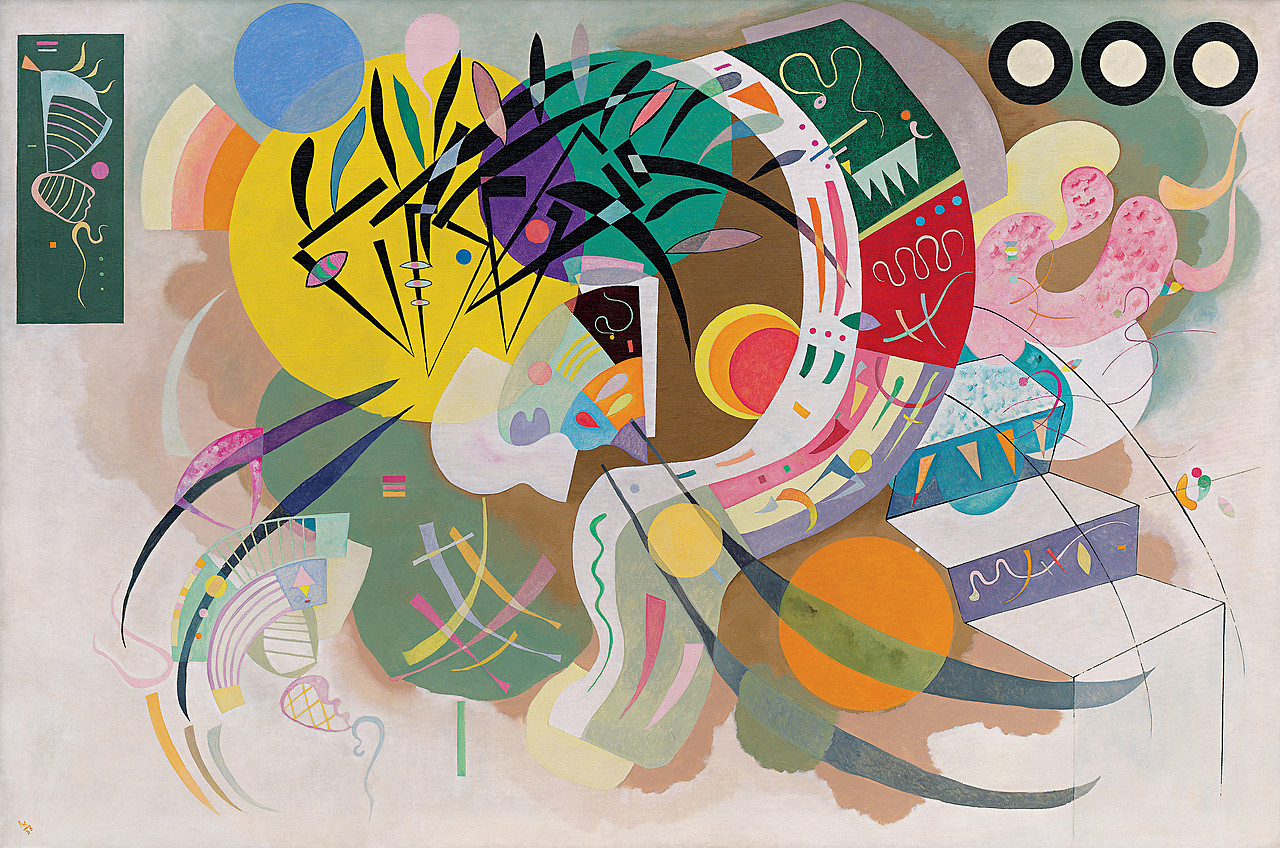This artwork, either an abstract painting or digital piece, is a vibrant explosion of colors and geometric shapes. The canvas is a rich tapestry of reds, greens, yellows, purples, blues, whites, blacks, beiges, and browns, blending together across various forms such as circles, triangles, rectangles, crescent moons, and squiggly lines. Dominantly, the image features a variety of circular shapes: a blue circle, an orange circle, a yellow circle, a multicolored circle of orange, yellow, and red, and a large yellow circle. There's also a near-perfect circle that is purple and green. 

On the left side, a dark green vertical rectangular box holds items that resemble harps—bearing lines of blue and pink. The painting’s background prominently features light gray and hints of gray-green hues. A ribbon-like or tapestry design flows across the middle with intricate patterns. Additionally, on the right, there’s a shape suggestive of stairs along with a partially donut-shaped form.

Although no text accompanies the artwork, the interplay of diverse shapes and colors creates a dynamic and engaging visual narrative, epitomizing the essence of abstract art where cohesion is eschewed in favor of visual interest and creative expression.